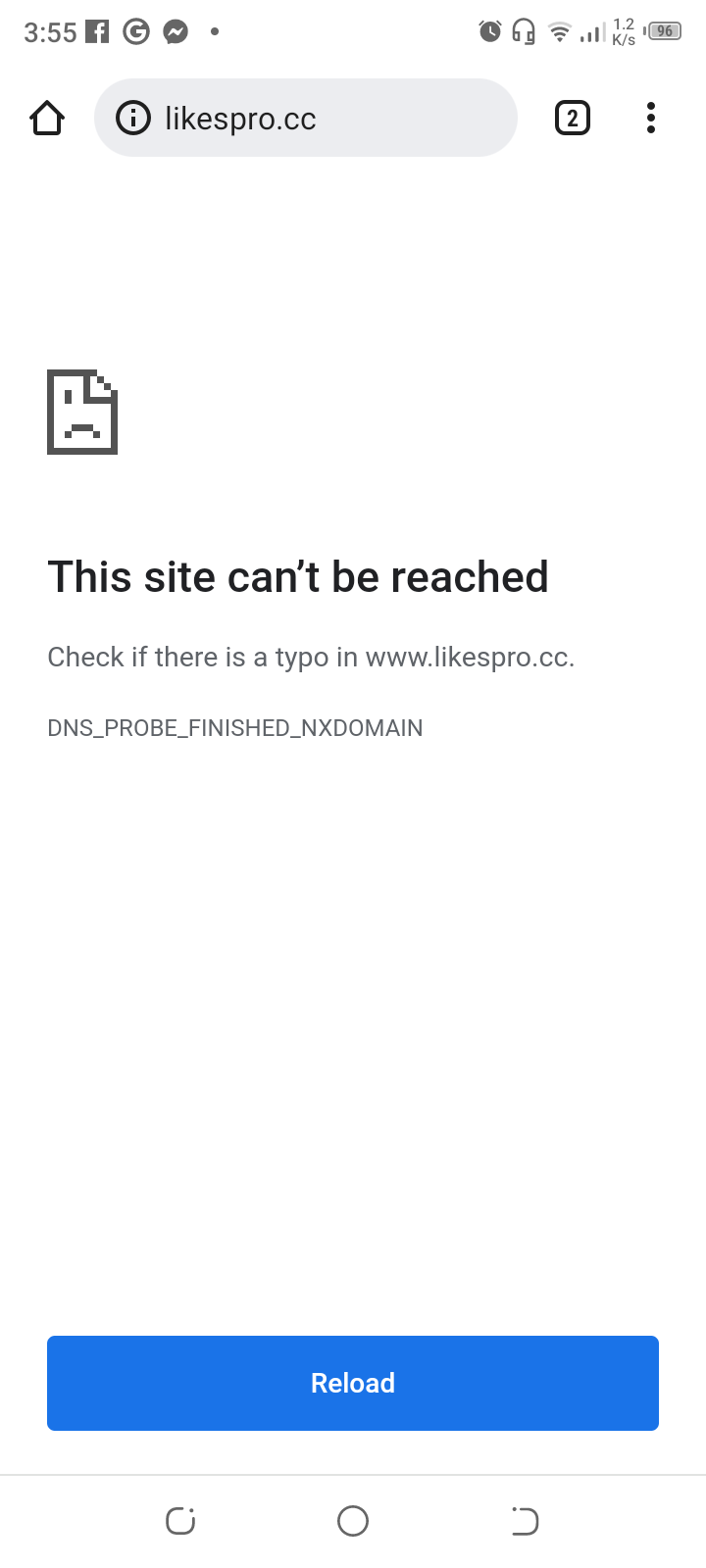This image is a detailed screenshot taken at 3:55, capturing someone’s attempt to access the website likespro.cc. At the top of the screen, we notice icons for Facebook, what appears to be Google, and Facebook Messenger. The URL in the search bar is clearly typed as likespro.cc, with a home button situated to the left of the search bar. To the right of the search bar, a square icon with the number 2 and a three-dotted line are visible. Additionally, there is an illustration of a piece of paper with a folded corner in the upper right side of the screen, featuring a single eye and a sad frown. The main message displayed prominently on the screen reads, "This site can't be reached." It advises checking for any typos in the URL, and further explains the issue with a note saying, "DNS_PROBE_FINISHED_NXDOMAIN." At the bottom center of the screen, there's a blue button labeled "Reload" in white text.